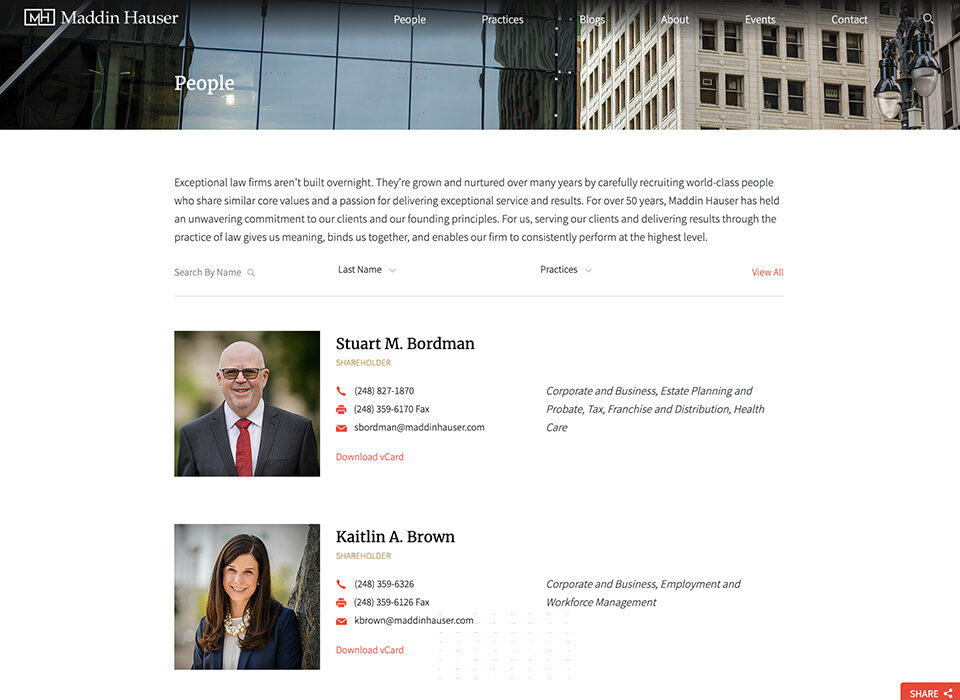The webpage belongs to Maddenhauser, prominently displaying their MH logo at the top. The navigation bar includes tabs labeled "People," "Practices," "Blogs," "About," "Events," and "Contact." Below the navigation, the focus is on the "People" section, featuring the text: "Exceptional law firms aren't built overnight. They are grown and nurtured over many years by carefully recruiting world-class people who share similar core values and a passion for delivering exceptional service and results. For over 50 years, Maddenhauser has held an unwavering commitment to our clients and our founding principles. For us, serving our clients and delivering results through the practice of law gives us meaning, binds us together, and enables our firm to consistently perform at the highest level."

The page includes a search box with the prompt "Search by name," filters such as "last name" and "practices," and an orange "View All" button. Below this section is a profile for Stuart M. Boardman, identified as a shareholder. His contact information includes a phone number, printer icon, mail icon, and a red "Download v-card" button. His practice areas are listed as Corporate and Business, Estate Planning and Probate, Tax, Franchise and Distribution, and Healthcare. An image of Stuart shows him in a suit with a red tie, white polo shirt, and glasses.

The second profile on the page belongs to Caitlyn A. Brown, also a shareholder. Her contact information is similarly structured with a download v-card button. Her practice areas are Corporate and Business Employment and Workforce Management. An image of Caitlyn depicts her in a blue jacket, white shirt, and a necklace.

The webpage's overall design features a white background with black text for clear readability.